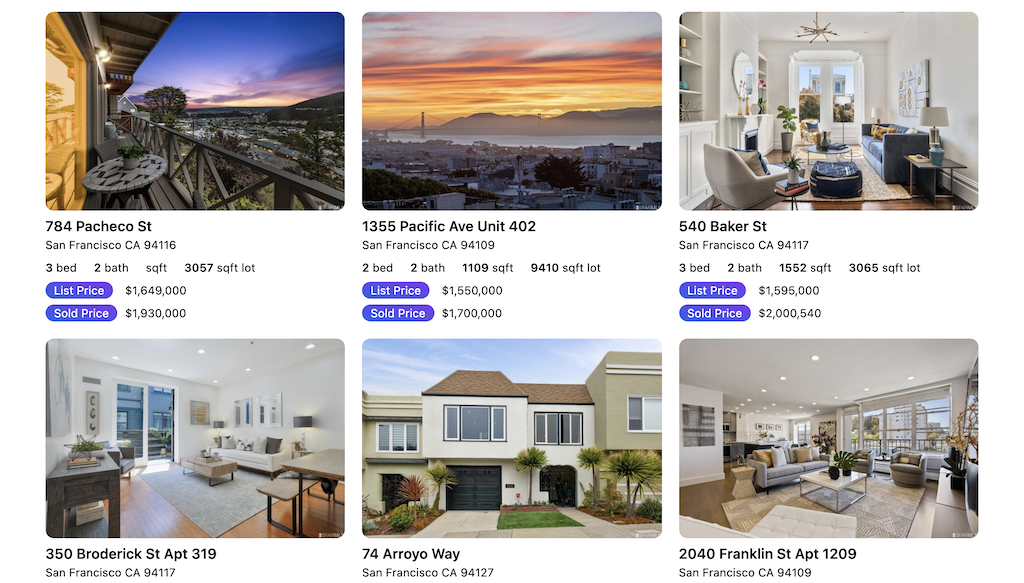A screenshot captures a section of a real estate website showcasing property listings. The snapshot features six property listings arranged in a 3x2 grid. Each property displays a photo, which could be an interior shot, an exterior view, or a scenic outlook connected to the home. Beneath each image, the specific address of the property is listed, followed by a line indicating "San Francisco, California" alongside varying zip codes.

For the properties in the top row, additional details are fully visible. These include the number of bedrooms, bathrooms, and the total square footage of the home. Directly below these details are two buttons: one purplish button labeled “List Price” with the corresponding price and another purplish button labeled “Show Price” adjacent to the actual listing price.

The bottom row of properties is partially cut off, showing only the address and city-line details without revealing information about bedrooms, bathrooms, or pricing.